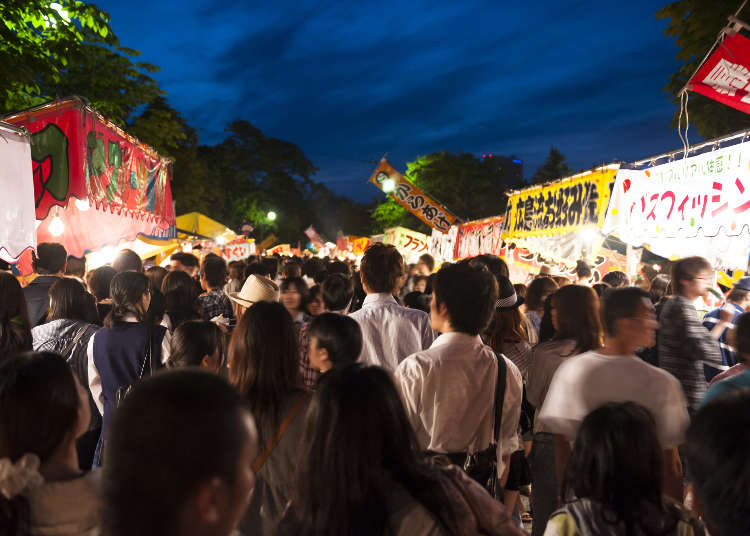The image captures a bustling scene at what appears to be a street market or festival in an Asian country, possibly China, given the language on the signs. The crowd is dense, with numerous individuals, men and women, moving in both directions, most with their backs towards the camera. Close to the camera, people with dark hair and carrying purses are noticeable. The atmosphere is lively and vibrant, enhanced by various brightly colored signs and banners on both sides of the alley. On the left, there's a red banner with writing, a yellow banner, and a brown sign protruding from a roof. On the right, a white banner with red letters is visible along with a yellow banner with black writing and an orange banner with black writing. The sky above indicates twilight, with dark clouds and lighter areas suggesting it is nearing night. Blue and red lights, possibly from an airport or building, are visible against the darkening sky, along with tall green trees in the background. Assorted lights from streetlamps add to the festive ambiance, emphasizing the crowded, energetic setting.